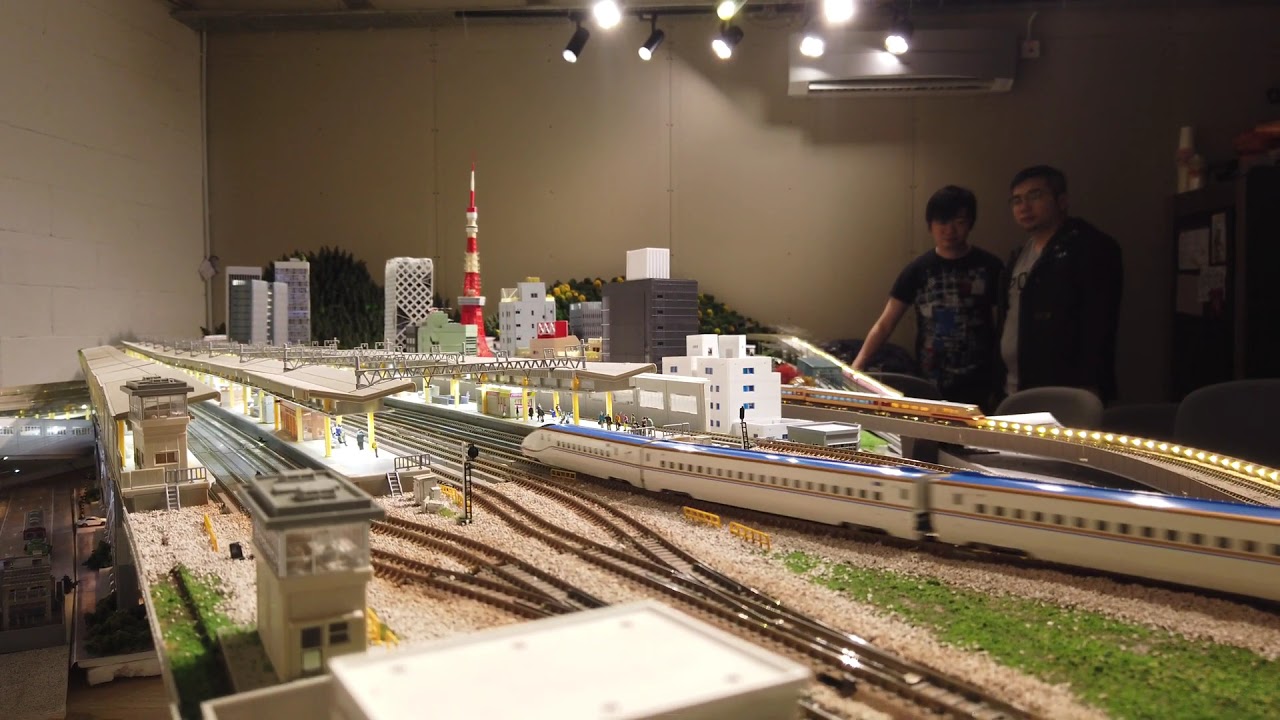This image showcases an intricate indoor model railroad set, positioned on a table approximately two to three feet high. The model features a white train with a blue top navigating two sets of converging tracks. The displayed scene includes an array of buildings, representative of a residential area complete with a tram station, signals, and a red and white tower. Inhabitants are depicted by small figurines populating the miniature community.

Overhead, eight distinct lights of various sizes and shapes illuminate the display. To the right of the central model, two younger men, possibly of Asian descent, observe the intricate setup. One of them seems to be wearing glasses, with a denim jacket layered over a white T-shirt, while the other dons a short-sleeve gray shirt with some design on the front.

The room's lighting casts a soft but detailed glow over the scene, while in the darker top-right corner, possible shelves or storage areas are visible. The primary colors featured in the model include off-yellow, tan, green, blue, white, and black, creating a vivid, lifelike miniature world.